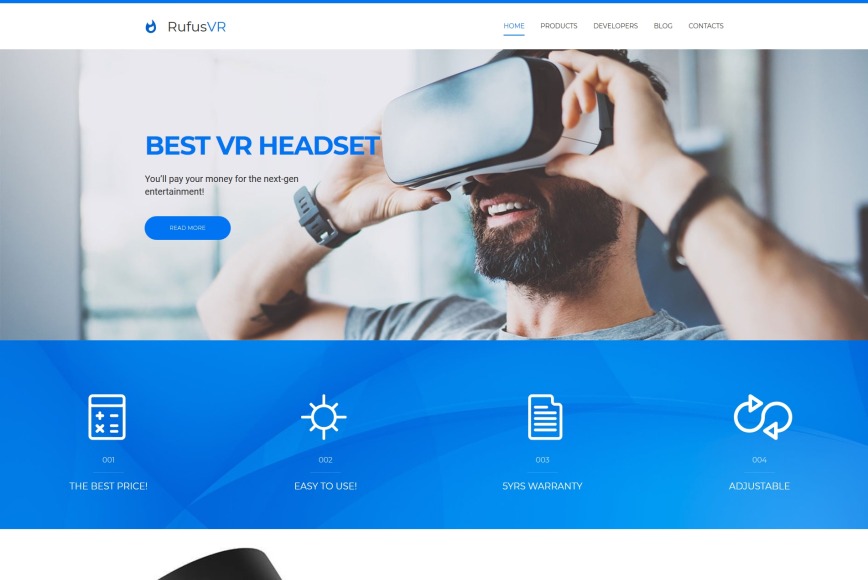This image is a computer screenshot in horizontal landscape orientation. At the very top, there is a thin blue bar. Below this blue bar, on a white background, the text "Rufus VR" is displayed from left to right, accompanied by a fire emoji. Further to the right on this white bar are navigation options: "Home" in blue, "Products," "Developers," "Blog," and "Contacts."

Beneath the white bar is a prominent image of a man using a VR headset. He is holding the headset up to his face with both hands. He has a watch on his right wrist and a bracelet on his left wrist. He is wearing a gray t-shirt, has a beard, and displays his teeth in a partially open mouth, revealing a hint of his nose. The man's hair appears to be brown, and there is a tattoo visible on his right hand. The background of this image is blurred, resembling a house or an office environment.

Below this image of the man are several sections. Firstly, a large blue bar takes up most of the lower portion of the image. This blue background features white icons and texts corresponding to different product features: 

- "001, Best Price" with an icon resembling a calculator
- "002, Easy to Use" with an icon that looks like a sun
- "003, SYRS Warranty" with an icon resembling a piece of paper
- "004, Adjustable" with an icon akin to an infinity symbol

Finally, at the very bottom of the screenshot is a block of white that contains a black bar, partially obscuring what appears to be an image, though details of this image cannot be discerned.